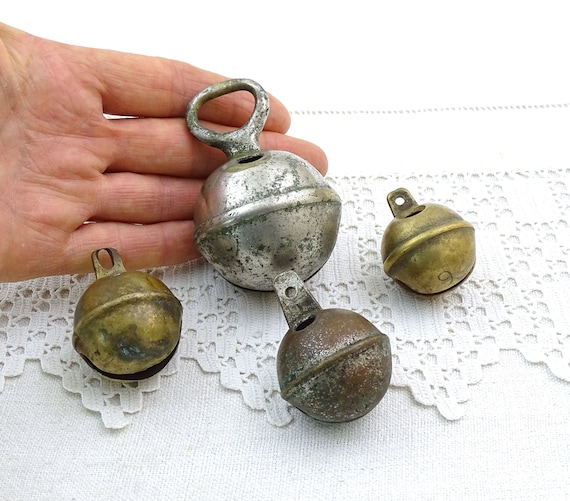In the image, an elderly, wrinkled hand extends into the frame from the left, cautiously holding a collection of ancient metal objects that appear to be fishing weights or possibly old Christmas tree ornaments. These objects vary in color; the most prominent one, positioned near the fingertips, shines with a silver hue despite its pitted and worn surface, evoking a chrome-like appearance. Surrounding it are three other similarly aged items: two on either side with a copperish-gold hue, and one more towards the bottom exhibiting a rusted, brownish color. Each item has a small hole at the top, suggesting they were once hung. The entire scene is set against a white background adorned with a quilted pattern, giving the image a delicate, old-fashioned ambiance. The overall appearance of these metal objects, with their textured and decayed surfaces, hints at a long and storied past, possibly underwater, imbuing the scene with a sense of antiquity and potential value.